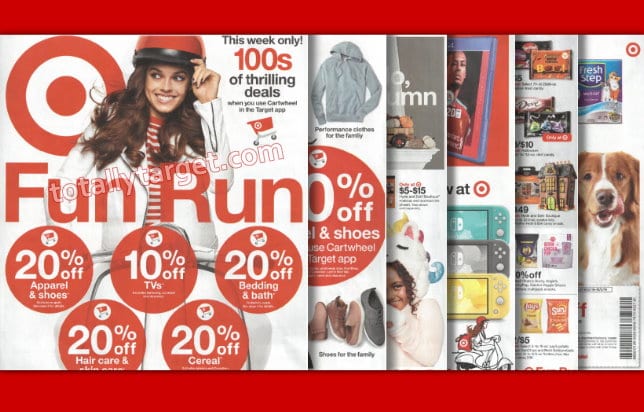The image features a promotional flyer from TotallyTarget.com. The flyer appears in a newspaper or magazine format typically delivered to homes. The main page is prominently displayed, with the TotallyTarget.com watermark visible.

The top and bottom of the page are bordered by red strips that span the width of the screen. The flyer bears the headline "Fun Run" in bold red letters on a white background, accompanied by Target's distinctive logo—a large circle enclosing a smaller one.

At the center of the flyer, there is a cheerful lady wearing a red helmet suited for scooter or motorbike riding. She is smiling and looking to the left, her long dark brown hair cascading down. She is dressed in a white and red striped t-shirt layered beneath a white, open long-sleeve jacket with a zipper. She is astride a white scooter, reinforcing the "Fun Run" theme. 

The top right corner of the page announces "This Week Only, Hundreds of Thrilling Deals," highlighting discounts including:
- 20% off apparel and shoes
- 10% off TVs
- 20% off bedding and bath items
- 20% off hair care and skin care products
- 20% off cereal

Behind the main page, five more pages are partially visible. They advertise various products such as shoes, clothes, electronics like Game Boys, and perhaps pet food, as suggested by the appearance of a dog on one page. Additionally, there is an image of a child in soft pajamas, indicating deals on children's apparel.